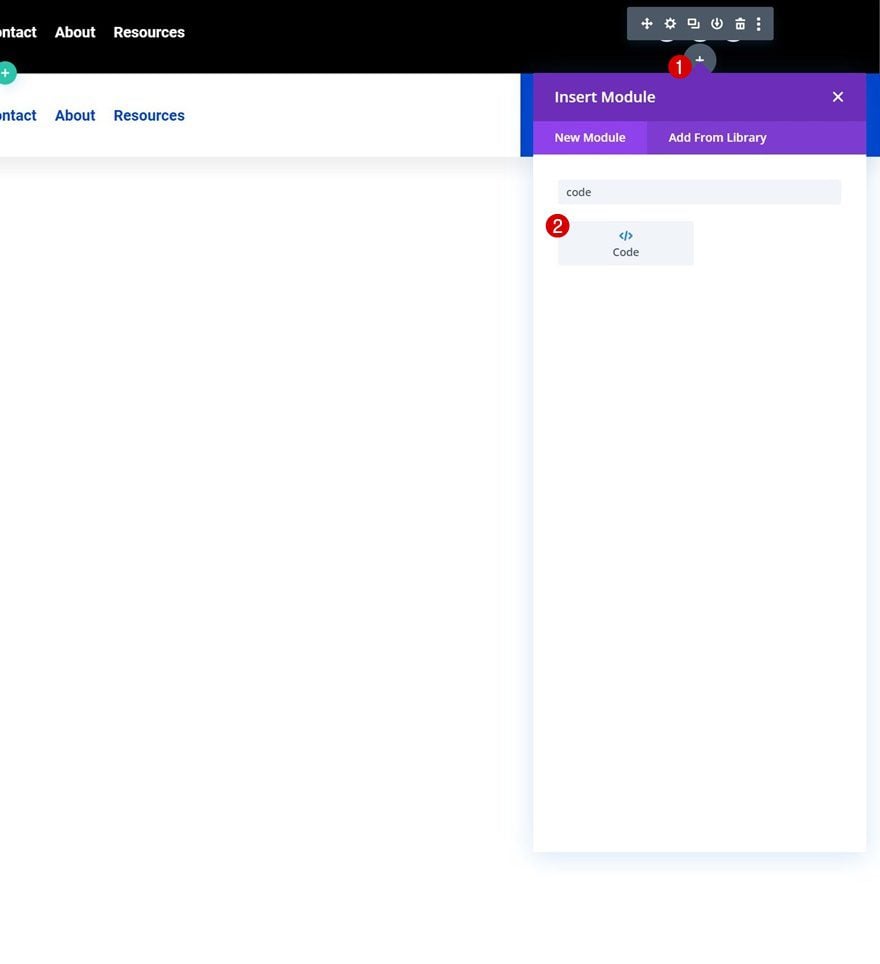This image captures a partial view of a website page, with about three-quarters of it visible. The top area features a black title or menu bar where the text partially reads "ntact," evidently the cut-off portion of "Contact." To the right of this are links labeled "About" and "Resources."

Below this black bar, there is an overlaid gray rectangle containing various icons: a plus sign, a settings gear, an on-off switch, and a trash can icon, presumably for deleting items. 

Further down, the left-hand side mirrors the top menu with another "Contact" link, suggesting a duplicate menu area. In this section, "Resources" is partially visible, and the background changes to white. 

Centered in this white area is a box labeled "Insert Module," set against a purple background. To the right of this box are options for "New Module" (highlighted) and "Add from Library." Within the "New Module" area, there appears to be a long rectangle box designated for inputting code. Beneath this, another box is labeled "Code," depicted with an arrow and a backslash icon, and features a red circle with the number "2" in one corner.